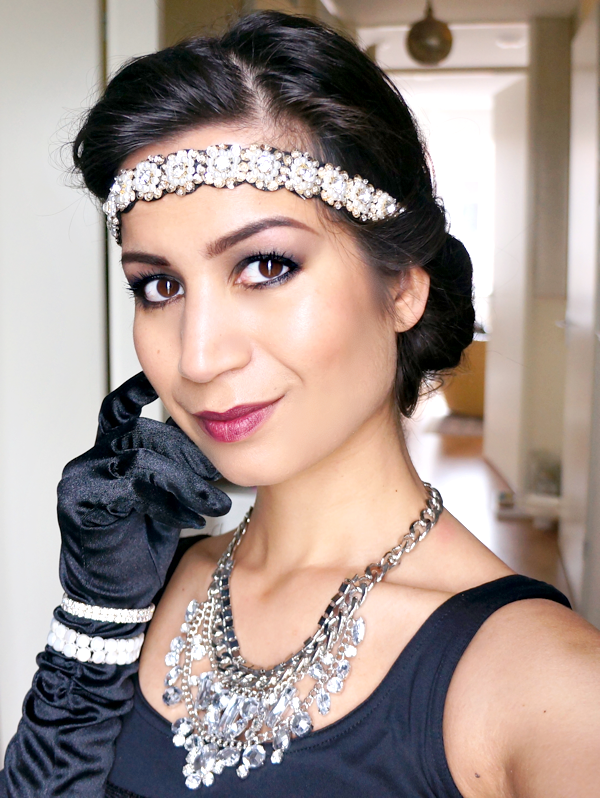The image depicts a young woman with slightly tanned skin and dark hair pulled back into a bun, giving her a refined and elegant appearance. Her heritage could be Middle Eastern, Italian, or Latina, as suggested by her complexion and features. She is smiling gently at the camera, her dark brown eyes framed by heavy eyeliner and complemented by purplish-red lipstick. She wears a striking, 1930s style ensemble consisting of a black strapped top with a U-shaped neckline and elbow-length black satin gloves. 

A jeweled headband, adorned with white floral-shaped rhinestones, rests gracefully across her forehead and extends behind her ears. Contributing to her opulent look, she dons a large, elaborate silver necklace with dangling diamonds and light blue accents. Her wrist is adorned with matching rhinestone bracelets over her gloves. The woman holds her gloved right hand up to her cheek, adding a touch of mystery and grace to her pose.

The background shows an indoor apartment setting with tan and light brown hues, suggesting wood floors, and featuring case openings, columns, and a round light fixture. Sunlight filters through a window, indicating it is daytime, while an open door adds depth to the scene. The woman fills the frame, visible from her chest to the top of her head and slightly angled with her left shoulder more forward, conveying an air of timeless elegance.